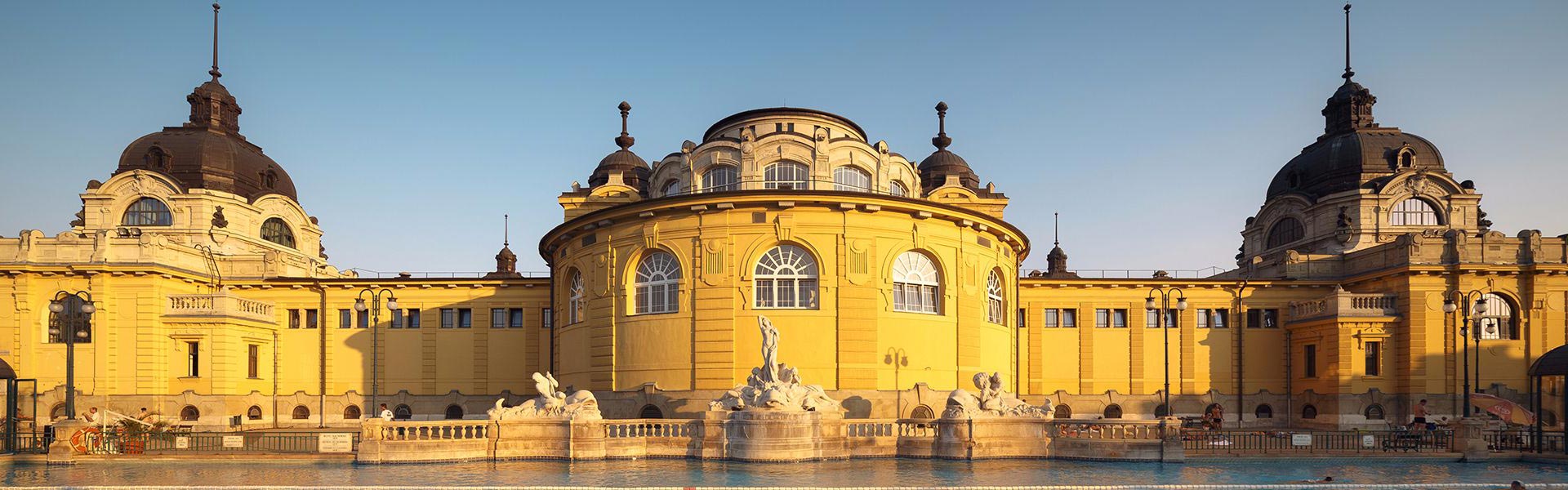The image depicts a long, narrow, yellow-brick building with a distinctly European architectural style, possibly a heritage site, shot during daytime under a clear blue sky. The structure features three prominent domes: a large central dome with a brown and cream-colored top, flanked by two smaller domes on either side. A concrete fence or barricade with heavy stone walls and pillars runs across the front, enclosing statues that appear to represent gods or goddesses. These statues, visible in front of the central dome, add a historic and cultural essence to the scene. White-trimmed windows punctuate the building's facade, and lamp posts are positioned around the area. In the foreground, a serene water body reflects the building, while people can be seen walking and resting, suggesting the site is frequented by tourists. The overall atmosphere is bright and sunny, enhancing the vivid colors and intricate details of this grand, elongated structure.